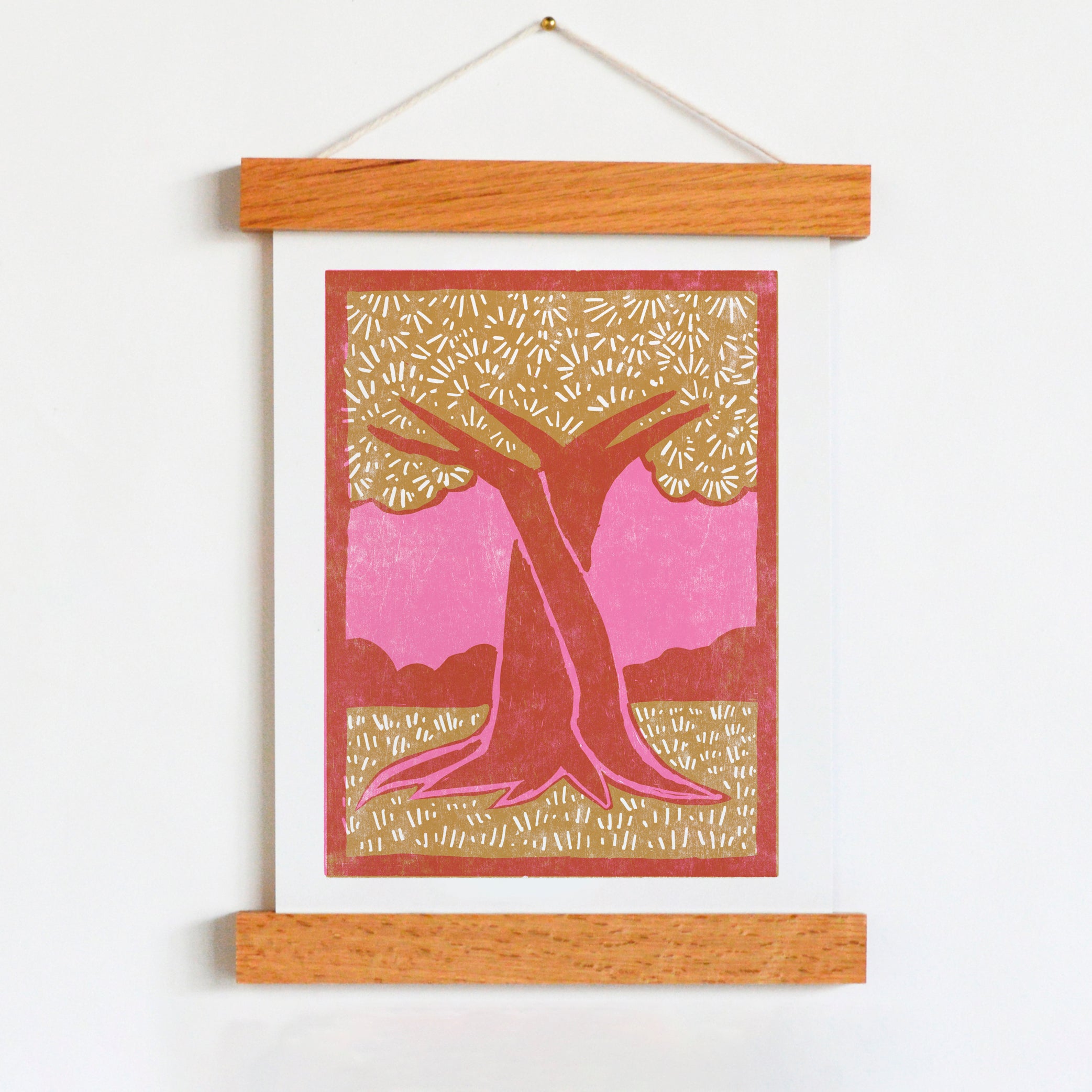The image depicts a painting of two intertwined trees in full bloom, set against a pink sky. The trees, outlined in reddish-brown and adorned with green leaves and white markings, rise from a base of green grass similarly accented with white. The painting is bordered by a red frame and mounted on a felt or paper material with a white border. The artwork is presented in a floating wooden frame with a string attached to a golden tack, which secures it flat against a white wall. The frame consists of a wooden plank at both the top and bottom of the painting, elegantly holding it in place. The overall color palette includes shades of pink, red, brown, green, and accents of white and gold. No text is visible on the artwork, and the setting appears indoors, though the specific location is not clear.